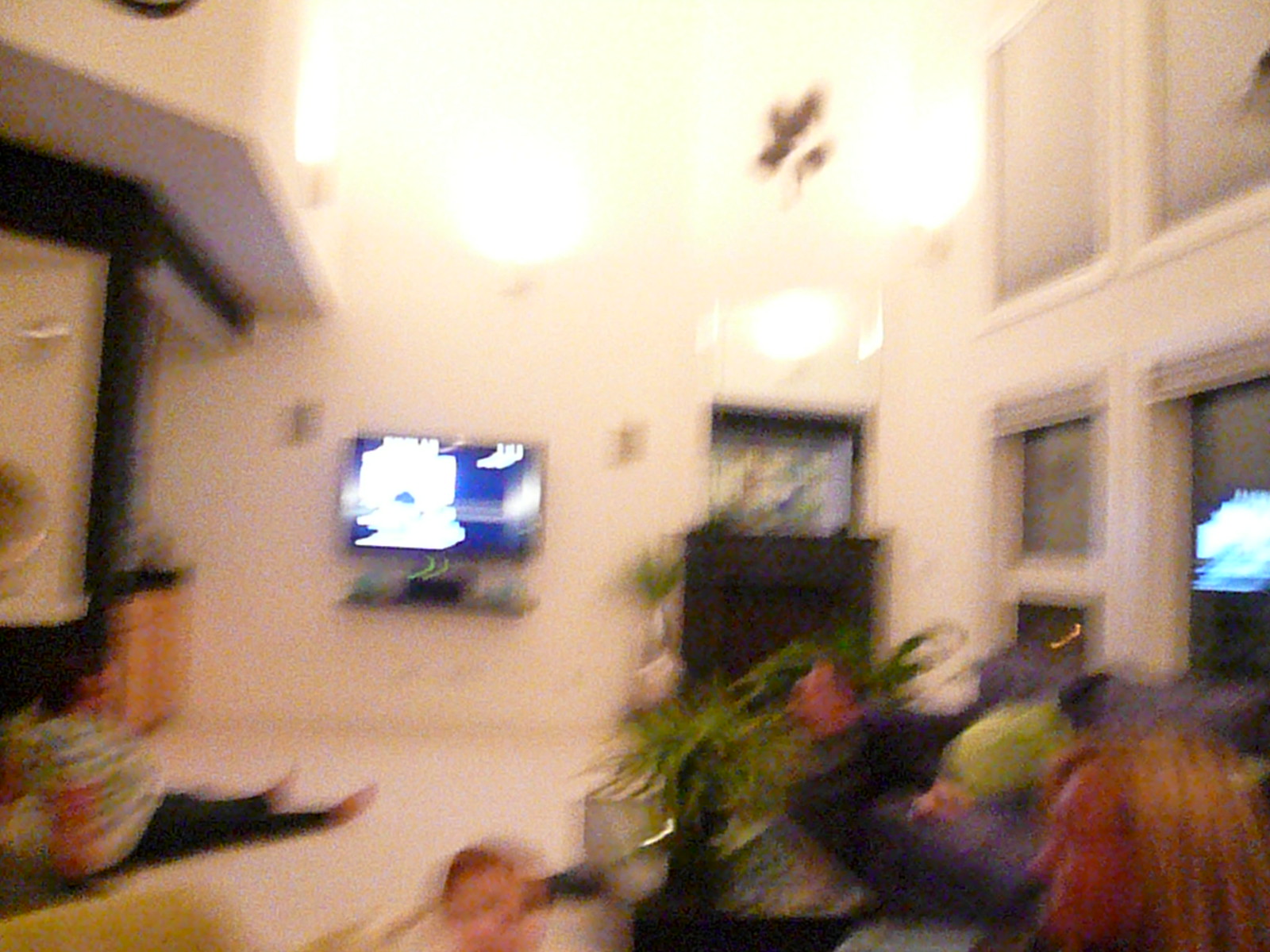This very blurry photo captures the scene inside a spacious living room with high ceilings and a large white wall at its center. The focal point of this wall is a relatively small TV flanked by light fixtures and two small gray speakers, with a shelf underneath holding some electronics. To the right of the TV, there is a black cabinet that seems to support a fish tank, with a light source positioned above it. Just next to this setup, there’s a green plant in a vase.

Occupying the left end of the room is a blue couch with a man reclining on it. In the bottom right corner of the image, partially visible, is the head of a woman with tanned skin and dirty blonde hair, who appears to be facing left. On a glass-surfaced coffee table nearby, there is another plant in a vase.

On the white carpeted floor, two children can be seen – one possibly crawling and the other lying down towards the bottom left-hand side of the image. Additionally, another person sits on the left side of the floor, legs extended straight out and arms bracing behind, facing the TV.

The living room also features large dark windows both at people height and higher up on the right side, adding to the airy feel of the room.